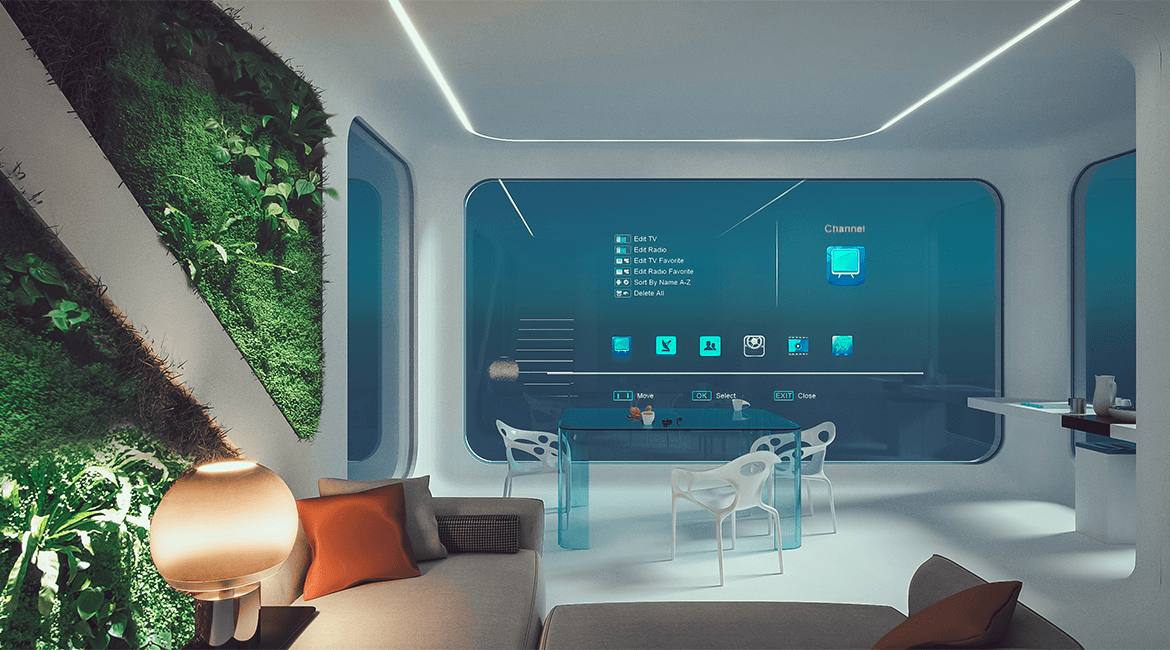The image depicts a highly detailed, computer-generated scene of a futuristic, science fiction-like room, which appears to be aboard a spaceship. The room has a sleek, white ceiling and gray walls. The far wall is split into two shades of blue—lighter on the top and darker on the bottom—resembling a computer screen displaying different icons and menus, including one labeled "channel" in white letters. On either side of this wall are large windows displaying blue screens without any visible content.

On the left side wall, there are two triangular cutouts filled with greenery, giving a natural touch to the otherwise high-tech environment. In front of these cutouts is a tan-colored couch adorned with pillows, along with a round lamp beside it. A glass table with three modern chairs is positioned centrally, enhancing the room's sophisticated atmosphere. Overall, the image skillfully combines elements of futuristic technology and indoor greenery to create a visually striking and immersive space.